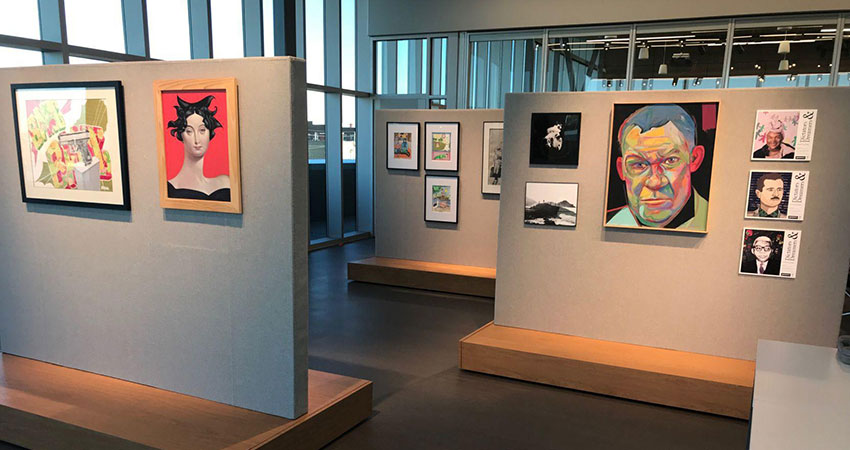The photograph depicts a section of a modern industrial art museum gallery, featuring various works of art on free-standing white walls with wooden bases against a background of large glass windows with vertical beams. The walls rise to approximately five feet six inches, guiding visitors through the exhibit. The room has wooden flooring that adds to its contemporary aesthetic.

In the foreground, a prominent white wall with a brown base showcases two distinct artworks. The first is a stylized portrait of a woman wearing a black hat and a black dress, set against a vibrant red background and framed in brown. Adjacent to this, a graphic design of a city street is displayed in a sleek black frame.

Towards the central section of the image, another white panel showcases six artworks. On the left, there are two smaller black-and-white photographs. In the middle, a prominently featured, pastel-colored portrait of a scowling gentleman wearing a white jacket and short dark hair. To the right, there are three vertical posters depicting different men, each with accompanying text, possibly depicting leaders from various countries. The backgrounds in these posters vary, with one being pink and the others being black.

In the background, a third panel stands between the others, this one set further back. It features four smaller artworks, all within black frames and white borders. Despite their distance, their vibrant colors and one partially obscured black-and-white photo hint at diverse subject matter and styles.

Overall, the image offers a glimpse into a thoughtfully arranged art gallery or museum exhibition, primarily showcasing stylized and abstract portraits, fostering a modern and engaging viewing experience.